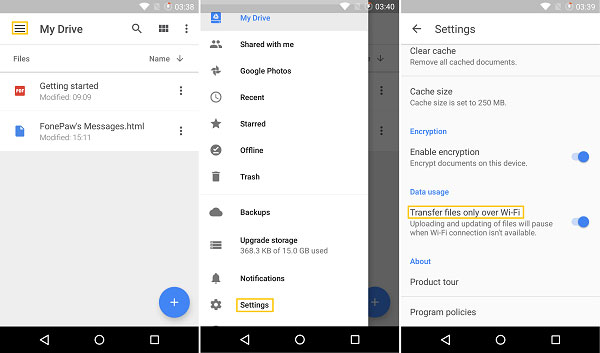This is a detailed printout of a "My Drive" page from a cloud storage service. 

On the left-hand side, there's a navigation pane that lists various categories: 
- "My Drive"
- "Files"
- "Shared with Me"
- "Google Photos"
- "Recent"
- "Starred"
- "Offline"
- "Trash"
- "Backups"
- "Upgrade Storage"

At the top of the "My Drive" section, under the "Files" category, we see an arrow pointing down next to "Name," indicating a dropdown menu for sorting. The displayed files include "Getting Started," last modified at 9:09, and "Messages.html," last modified at 15:11.

In the middle section, a summary bar informs that 368.3 KB of 15.0 GB storage is used. It also includes options for "Notifications" and "Settings."

On the far right, under the "Settings" category, there's a detailed list with another arrow pointing left. The settings listed are:

- "Clear Cache": an option to remove all cached documents.
- "Cache Size": currently set to 250 MB.
- "Encryption":
  - "Enable Encryption"
  - "Encrypt Documents on this Device"
- "Data Usage":
  - "Transfer Files only over Wi-Fi": stating that uploading and updating files will pause if Wi-Fi isn't available.
- "About":
  - "Product Tour"
  - "Program Policies"

Next to both "Enable Encryption" and the "Data Usage" options, there are two blue buttons indicating these settings have been activated.